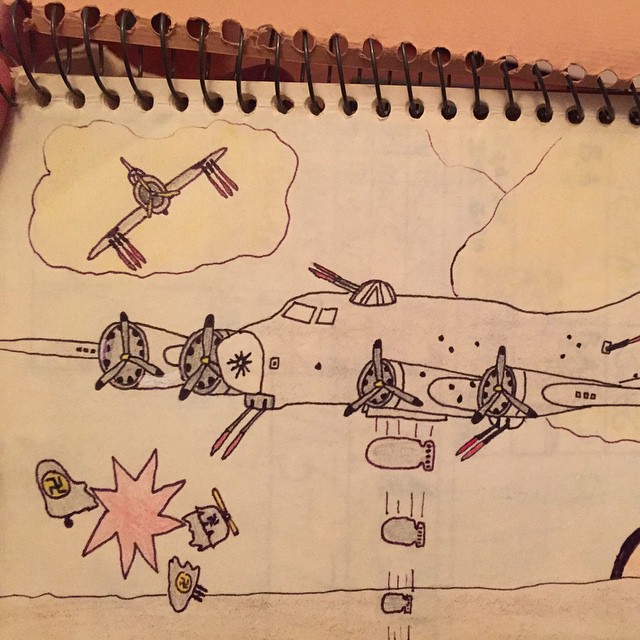The image is a hand-drawn depiction of a wartime scene, likely created by a child. It features two airplanes engaged in combat, rendered in black pen on a white sheet of paper from a note binder, with visible metal rings. One of the planes is dropping bombs, surrounded by clouds and a rough outline of the ground below. The other plane, marked with a swastika, appears to be exploding, suggesting a World War II context. The paper shows parts of the binder, which is made of brown, almost cardboard-like material. The planes exhibit additional details such as arrows stuck in one of them, indicating damage, and the presence of a red missile being launched. Yellow and red colors accentuate parts of the aircrafts, emphasizing the chaotic nature of the air battle.